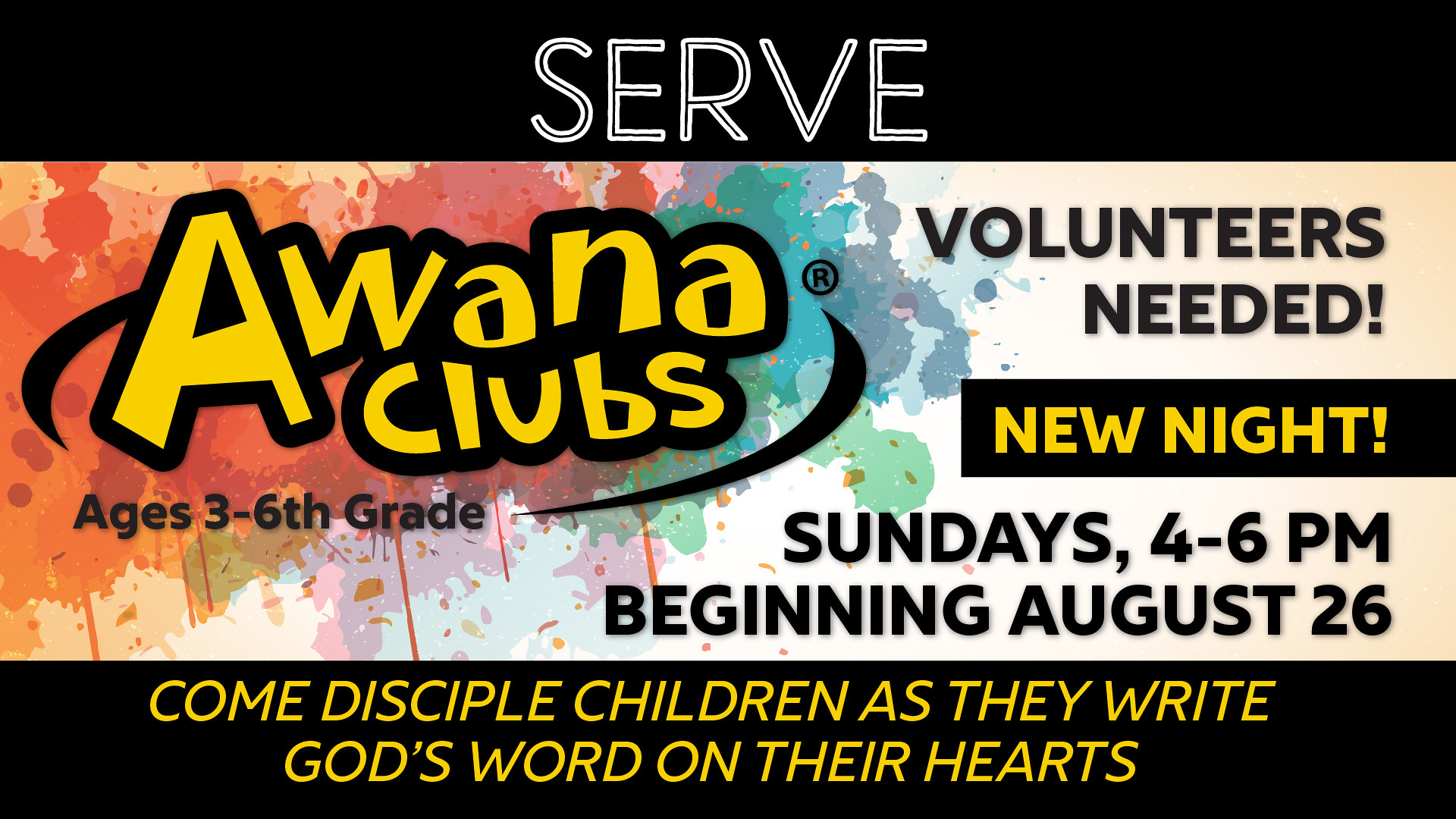This image is a colorful digital poster advertisement. At the top, there is a black horizontal strip featuring the word "SERV" in white letters. The center background consists of vibrant paint splashes in various colors, including red, orange, green, blue, and purple. Overlaying this colorful background is text in yellow and black that reads: "Awana Clubs, ages 3-6th grade. Volunteers Needed. New Night: Sundays 4-6 p.m., beginning August 26." Towards the bottom of the image, another black horizontal strip contains the text in bright yellow: "Come disciple children as they write God's word on their hearts." The poster effectively uses a mix of bold colors and contrasting text to emphasize its call for volunteers and promote the event details.